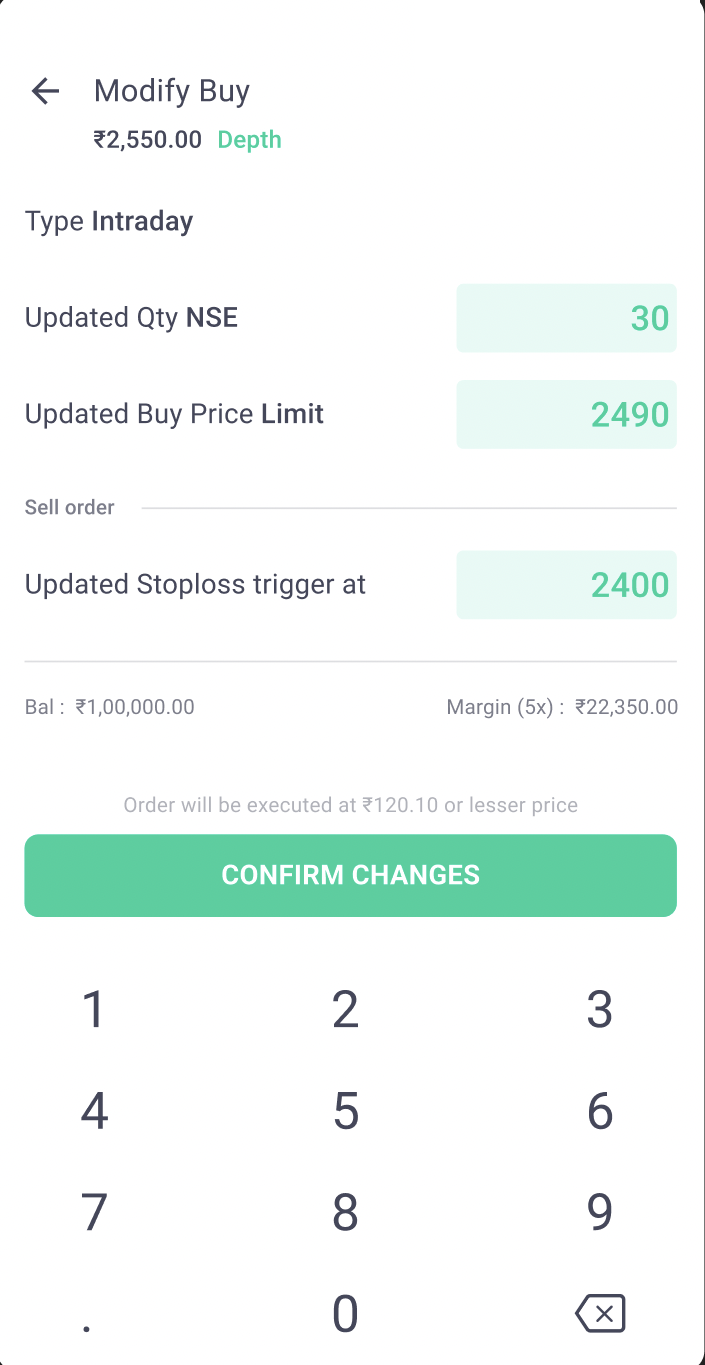The image depicts a mobile phone screenshot of a financial trading app. The interface features a white background with black text and green highlights. At the top, there is a back arrow followed by the title "Modify Buy." Directly below this title, the amount €2,550 is displayed along with a green link labeled "depth." Further down, the page details "Type: Intraday" showcased by "Quantity: 30" and "Price Limit: 2490." Additionally, a "Stop-Loss Trigger" is set at "2400." A prominent green button labeled "Confirm Changes" appears towards the bottom of the screen. Beneath this button, a numeric keypad is visible, indicating the app is ready for further input. The concise, structured layout ensures users can quickly review and adjust their trading parameters.